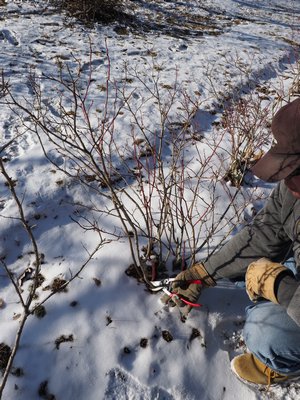In this detailed winter photograph, a man is captured outside on a partially snowy ground, crouched beside a leafless shrub. The man is wearing a dark gray jacket, blue jeans, light brown boots, tan gloves, and a brown hunter's cap. He is positioned on the right side of the image, focused on pruning one of the shrub’s stems near the roots with a pair of red-handled pruners. Despite the chill of the season, it's a sunny day, with the sunlight casting long shadows across the patchy ground where melting snow reveals patches of dirt. In the background, there are animal tracks dotting the snow, and further shadows stretch across the scene, possibly from a tree or pole. The bare shrub, centrally located, starkly contrasts with the wintery setting, emphasizing the man’s meticulous gardening efforts even in this cold season.